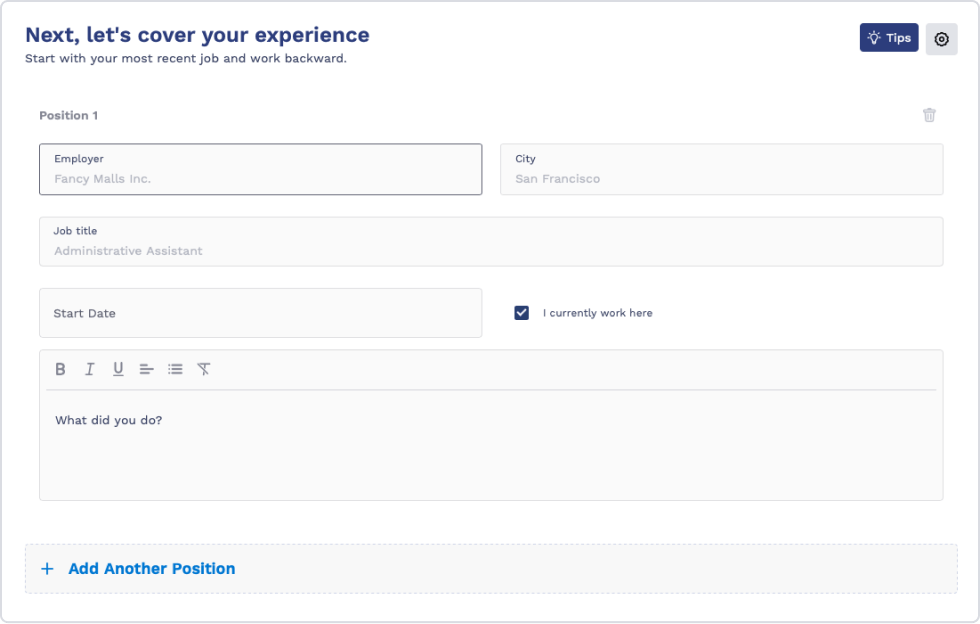The image is a detailed screenshot from a computer screen, displaying a section of a job application or resume-building interface. The interface has a large, rectangular layout with a white background transitioning to blue at the top. At the top-center of this section, bold text reads, "Next, let's cover your experience."

On the far right side of this header is a blue button labeled "Tips," alongside a small gray square with a gear icon, indicating settings or additional options. 

Below the main heading, instructional text advises, "Start with your most recent job and work backward."

The interface lists a job position with the title "Position 1." For this position:
- The employer is specified as "Fancy Malice Incorporated."
- The location is noted as "San Francisco," adjacent to the right.
- The job title is "Administrative Assistant," located beneath the employer name.

A long, gray box labeled "Start Date" remains blank, awaiting input. To the right of this, a check box labeled "I currently work here" is ticked.

Further down, a prompt box titled "What did you do?" invites the user to describe their responsibilities and achievements.

At the bottom of the section, a prominently displayed, long, skinny, gray rectangular button with a blue plus sign and the text "Add another position" encourages the user to input additional previous job roles.

The overall design and instructions suggest that the individual is either applying for a job or constructing their resume.